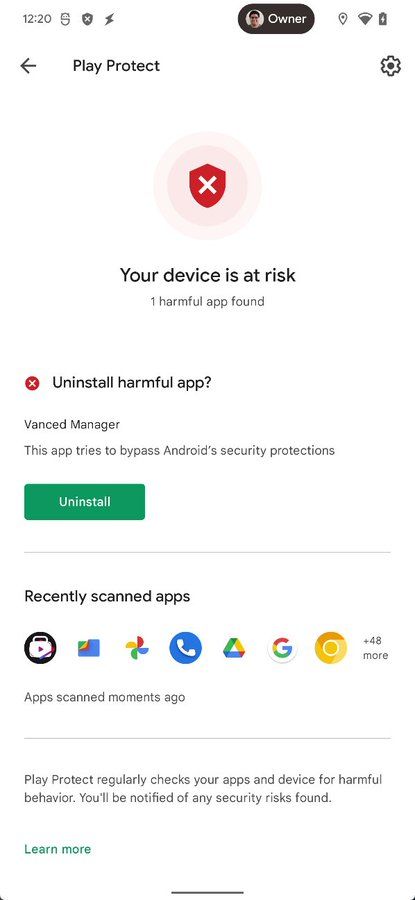Screenshot of a cell phone screen displaying a security alert from the Android operating system. The screen has a white background, and at the top, the time and date are visible along with the phone owner's name and profile picture. Prominently featured in the top-middle section is a red shield icon encircled by pink rings, with an "X" symbol inside the shield. Directly below the shield, the message "Your device is at risk, one harmful app found" is displayed.

The alert then prompts the user to either "Uninstall the harmful app" or "Go to your advanced manager." It warns that the detected app attempts to bypass Android's security protections, confirming the device is running on an Android platform.

Further down the screen, there is a section showing icons of recently scanned apps, followed by a message from "Play Protect" stating, "Regularly check your apps and device for harmful behavior. You'll be notified of any security risks found." At the bottom of the alert, a green button is provided for the user to click and uninstall the harmful app, emphasizing the importance of addressing the security risk.